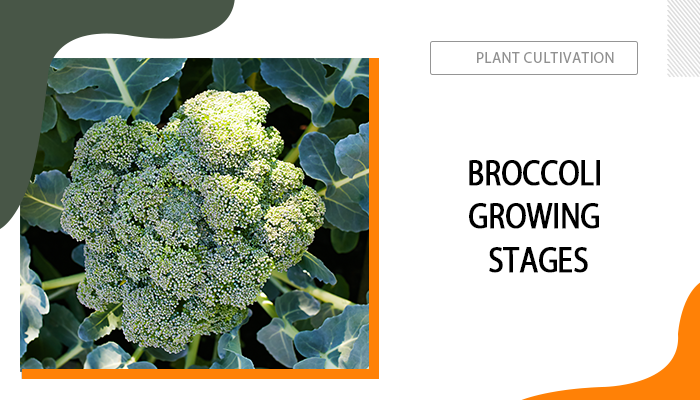The image is a detailed visual presentation focusing on broccoli within a bifurcated layout. A photograph of green broccoli, featuring its florets and leaves, is prominently situated in a square inset on the left side of the image. The broccoli is framed by an orange border along the right side and bottom. This photograph appears to be taken in sunlight, adding vibrance to the green hues of the broccoli and its surrounding leaves. The background of the image is white.

On the right side of the image, at the top, a rectangular box contains the text "Plant Cultivation" in gray font. Below this, in large black capital letters, it states "BROCCOLI GROWING STAGES." The corners of the image are accentuated with a design element; the top left corner has a grey motif while the bottom right corner displays an orange section, which aligns with the orange border framing the broccoli photograph. The overall setting and style emphasize vegetables, presenting a clear, educational slide about broccoli cultivation stages.